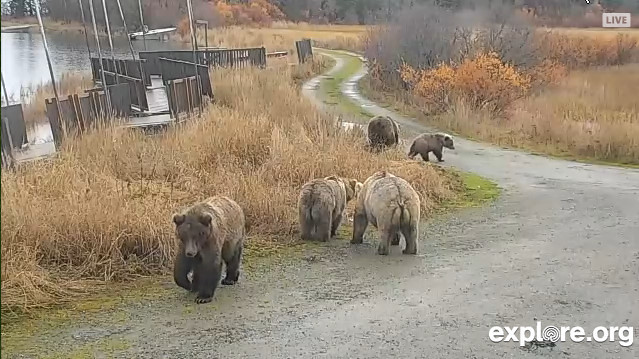The photograph captures a rural scene featuring five brown bears with dark brown coats near a winding gravel road that cuts through a golden-brown field. The overcast sky casts a muted light over the landscape, emphasizing the autumn hues. The road, light gray from pulverized gravel, meanders through fields of varying foliage: golden strands of grass, orange bushes, and patches of light green and brown foliage. To the left of the road, there are taller brown plants and a wooden walkway with chocolate-brown railings. On the right, a pond with light and dark gray waters is bordered by trees in transitions of orange, yellow, golden, and bare branches. The bears are scattered along the road, with three closer to the camera and two further down the path. The bottom right corner of the image features a watermark reading "explore.org," with the letter 'O' replaced by a logo, and the top right corner has a "live" indicator in a gray square, signifying a live broadcast.